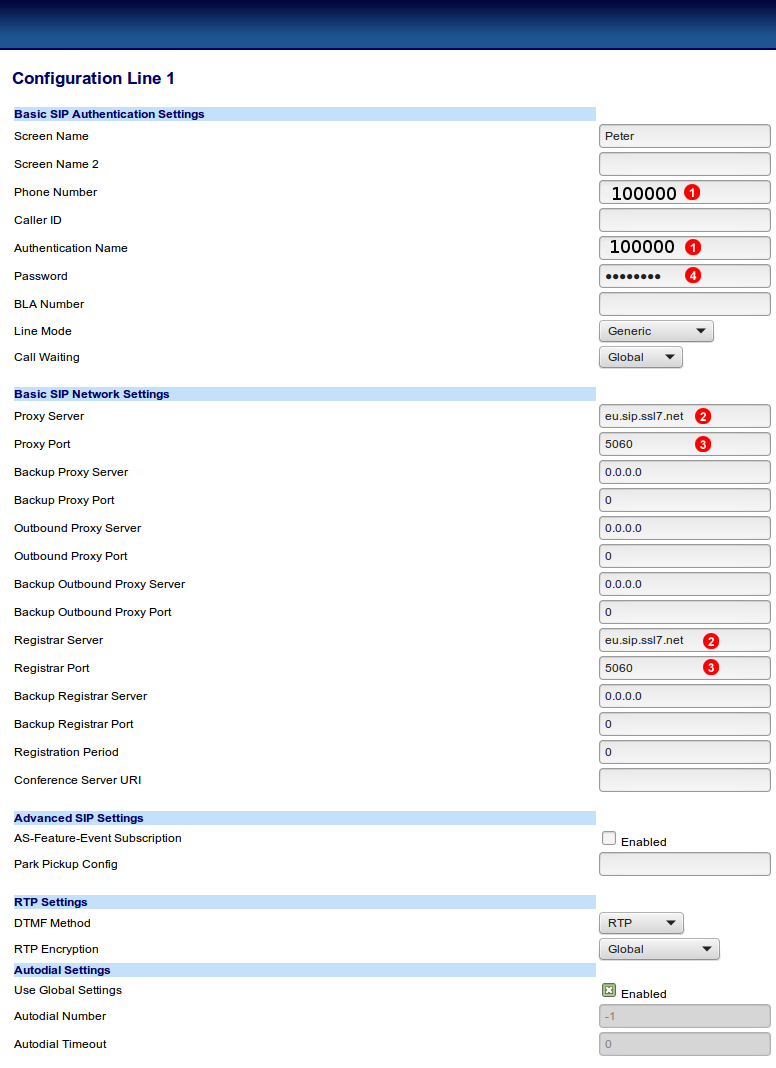### Detailed Caption for SIP Configuration Web Page Screenshot

The image displays a web page interface for configuring SIP (Session Initiation Protocol) settings, characterized by a blue bar at the top. 

#### Basic SIP Authentication Settings:

- **Screen Name:** Unspecified
- **Phone Number:** 100,000 (highlighted with a red '1')
- **Caller ID:** Blank
- **Authentication Name:** 100,000 (highlighted with a red '1')
- **Password:** Obscured, indicated by a series of dots, with a red '4' next to it
- **BLA Number:** Blank
- **Line Mode:** Generic
- **Call Waiting:** Global

#### Basic SIP Network Settings:

- **Proxy Server:** eu.sip.ss17.net (highlighted with a red '2')
- **Proxy Port:** 5060 (highlighted with a red '3')
- **Backup Proxy Server:** 0.0.0.0
- **Backup Proxy Port:** 0
- **Outbound Proxy Server:** 0.0.0.0
- **Outbound Proxy Port:** 0
- **Backup Outbound Proxy Server:** 0.0.0.0
- **Backup Outbound Proxy Port:** 0
- **Register Server:** eu.sip.ssl7.net (highlighted with a red '2')
- **Register Port:** 5060 (highlighted with a red '3')
- **Backup Register Server:** 0.0.0.0
- **Backup Register Port:** 0
- **Registration Period:** 0 seconds
- **Conference Server URI:** Blank

#### Advanced SIP Settings:

- **Feature Subscription Enabled:** Not checked
- **Pickup Park Configuration:** Blank
- **DTMF Method:** RTP (Real-time Transport Protocol)
- **RTP Encryption:** Global
- **Auto Dial Settings:** Enabled (using global settings)
  - **Auto Dial Number:** -1
  - **Auto Dial Timeout:** 0 seconds

This web page is likely used for setting up a phone server or a personal SIP server, providing detailed configurations for authentication and network settings.